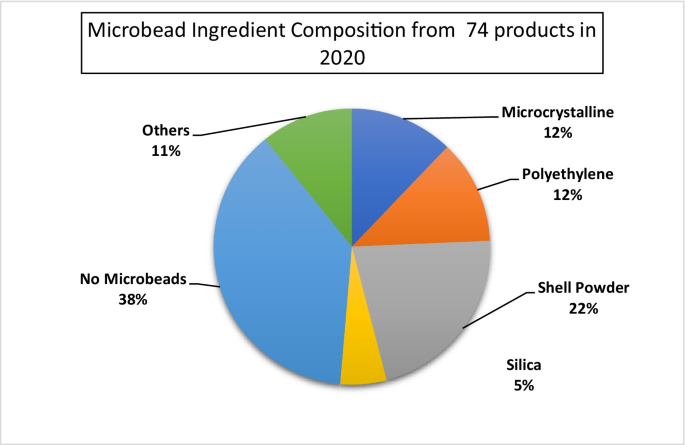The image is an illustrative pie chart displayed against a plain white background with all accompanying text in simple black font. At the top of the image, there is a header framed by a black rectangle that reads, "Microbead Ingredient Composition from 74 Products in 2020." The pie chart itself is prominently centered and divided into six distinct colored slices, each representing different ingredients. The largest slice, colored light blue, indicates that 38% of the products contain no microbeads. Adjacent to it, a green slice represents 'Others' at 11%. A darker blue slice, labeled 'Microcrystalline,' makes up 12% of the chart. Another 12% is accounted for by 'Polyethylene,' illustrated in dark orange. 'Shell Powder' is shown in a gray slice, comprising 22% of the total. The smallest slice is colored yellow and represents 'Silica,' making up 5%. Each slice is accompanied by black text specifying the ingredient it represents and its corresponding percentage.